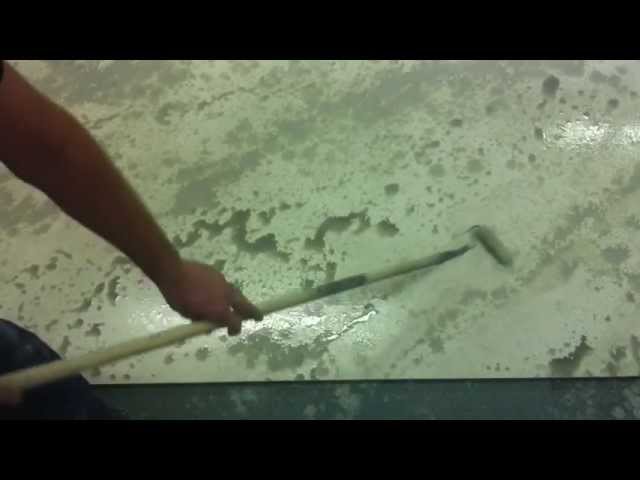The photograph captures a person using a paint roller attached to an extended pole, presumably with both hands, though only their left arm is visible from the left side of the image. The pole is exceptionally long and extends downwards, reaching a stone or concrete floor that features green splotches or dirty water. The roller appears to be applying or spreading this watery substance across the floor. The scene is framed with black bars at the top and bottom, indicating some cropping of the original image.